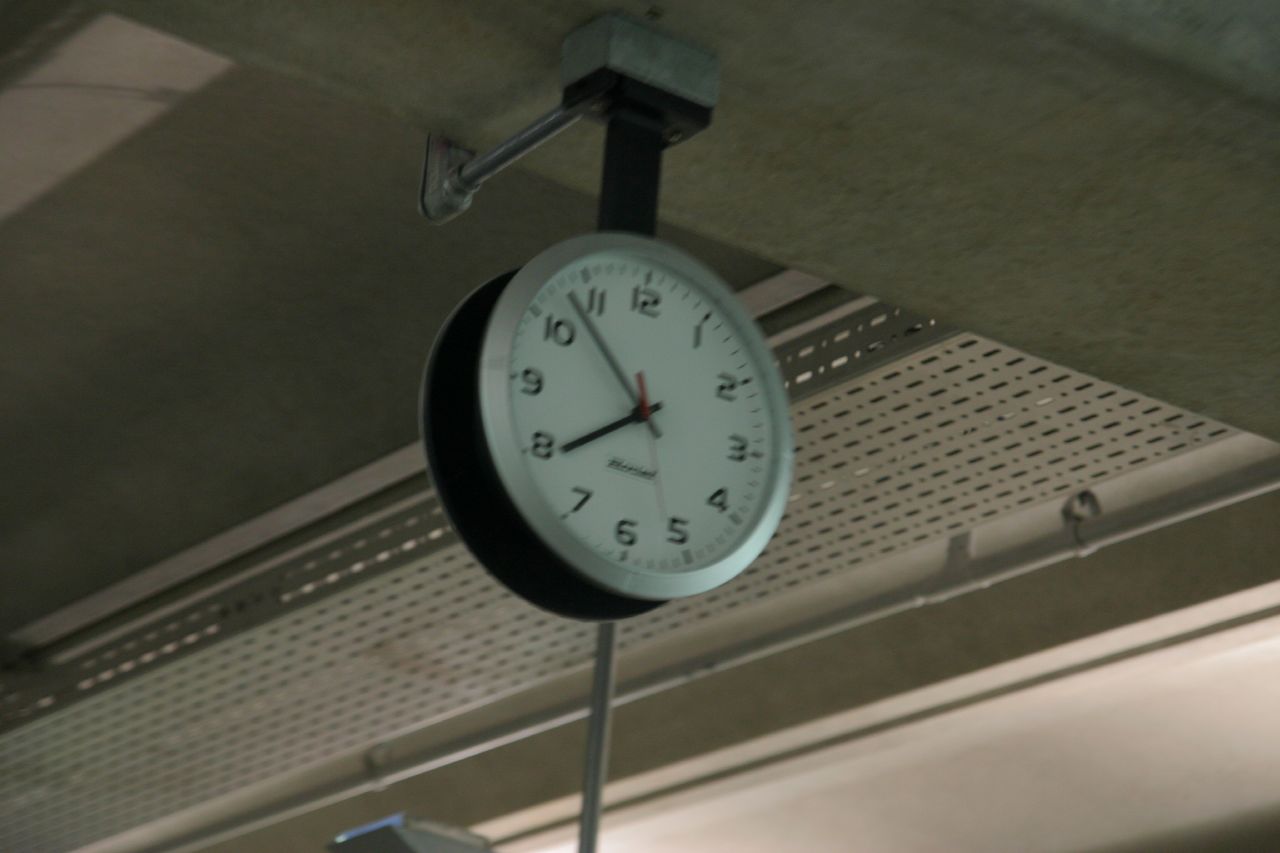The image showcases the interior of an industrial-style building from a low-angle perspective, giving the impression of looking upwards. Dominated by large concrete beams and walls in tan and gray hues, the ceiling features an intricate arrangement of beams—some are gray and others white, adorned with evenly spaced tiny holes. The play of light and shadows cast across the ceiling suggests a light source is creating varying brightness levels throughout the space. 

Prominently, a silver object protrudes from one of the white beams, although its exact purpose isn't clear due to the limited context provided by the tight framing. Further below, intersecting with the concrete beam, is a silver component connected to a black element, ultimately culminating in a circular black fixture. Suspended from this fixture is a clock, distinguished by its silver rim, white face, black hour and minute hands, and a red second hand. The clock is attached and appears to be hanging down from the ceiling or wall, adding a functional and aesthetic element to the otherwise stark industrial environment.